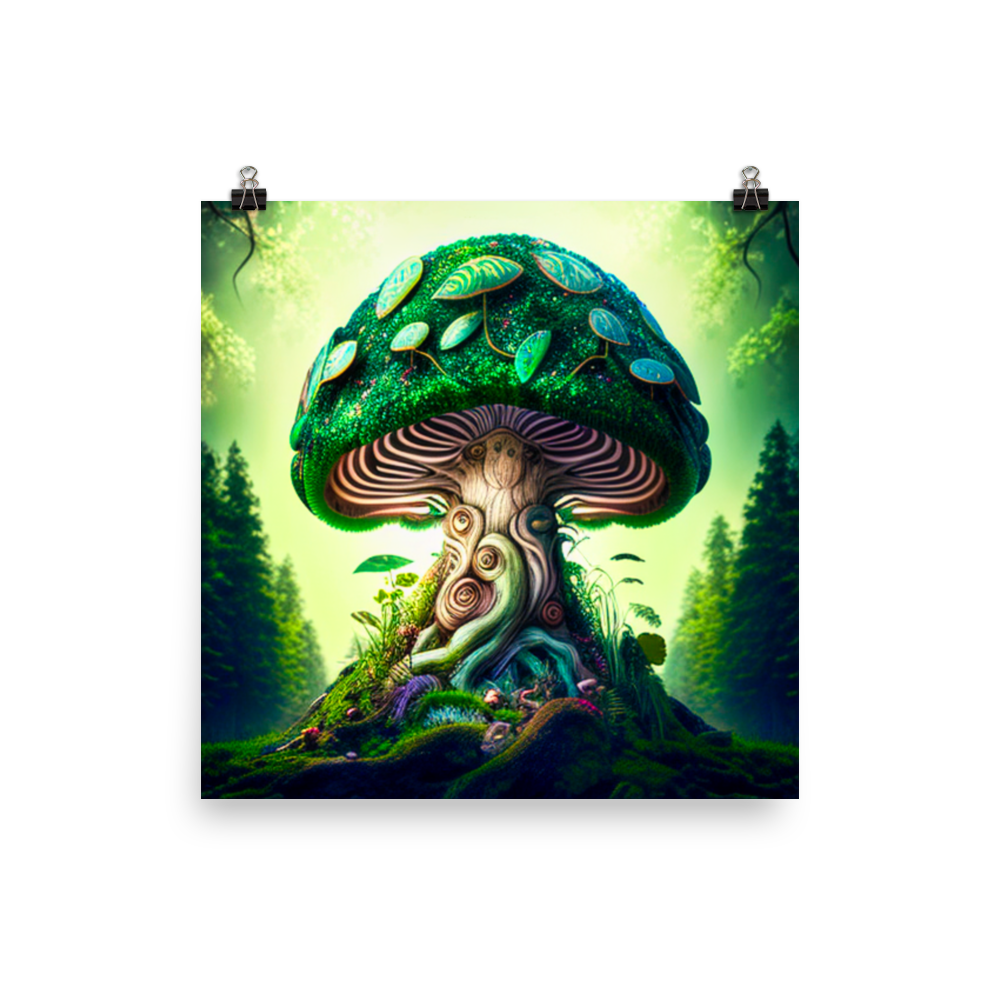This detailed, computer-generated artwork depicts a larger-than-life green mushroom emerging from lush, mossy soil amidst a field framed by blurred, dark green pine trees. Illuminated by sunlight beams, the mushroom, which combines organic and fantastical elements, captivates with its intricate design. The cap is adorned with moss, leaves, and a foliage-like rounded top, and features the distinctive ribbing of mushrooms as well as white and black stripes on its underside. The stem is a vibrant amalgamation of swirling, multicolored patterns and various root shapes, woven with decorative swirls transitioning from cream to green to blue. Embedded in the stem are hints of faces and a creature-like form with two eyes and arms that seem to support the mushroom cap. The scene is whimsically detailed with additional foliage and moss-covered roots, while in the shadow on the right, a human figure rests against the mushroom, adding a touch of surrealism to the mystical landscape. The artwork is held up by two clamps at the top, set against a white background.